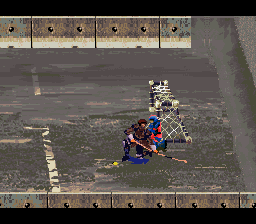This image appears to be a pixel art screenshot of an old-school video game, depicting a street hockey scene set in an urban environment. The action takes place on a worn, gray concrete surface, indicated by textures that mimic dirt and lines suggesting parking spaces or lanes. Two figures are central to the scene: one dressed in a brown-burgundy outfit and the other in a red-blue ensemble. Both are kneeling and wielding hockey sticks, appearing closely together as they face off near a hockey goal net positioned to the left-center of the image. The scene is framed by cement pillars and bolted walls on either side, reinforcing the gritty, urban atmosphere.